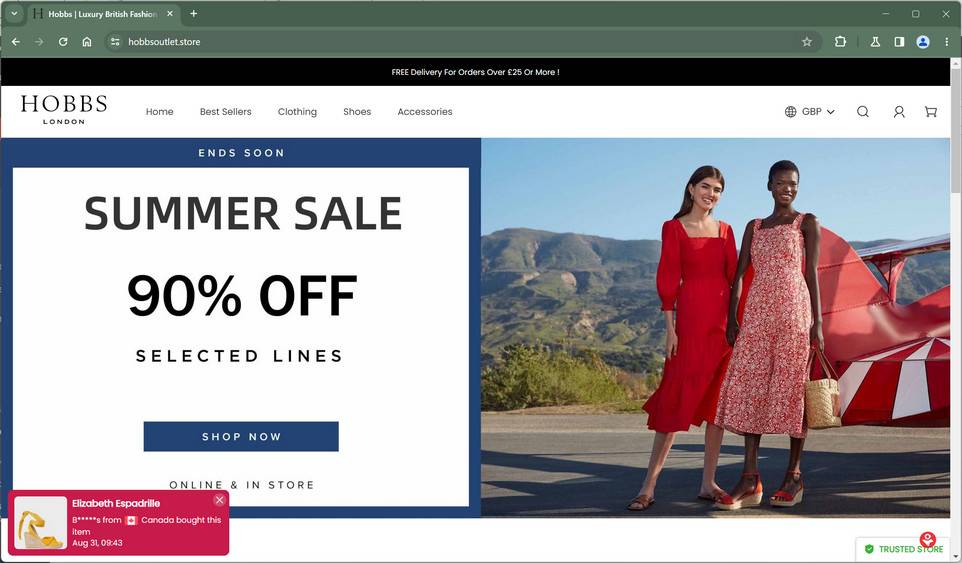The website for Hobbs London features a forest green top banner prominently displaying the Hobbs Outlet search bar. Directly beneath, a sleek black banner announces "Free delivery for orders over £25" in striking white text. Under this, the Hobbs London logo appears alongside navigation tabs labeled 'Home', 'Best Sellers', 'Clothing', 'Shoes', and 'Accessories'. To the right, there are icons for search functionality, cart access, and user login.

Further down, a vibrant announcement declares "End Soon: Summer Sale, 90% Off Selected Lines" with a "Shop Now" button indicating availability both online and in-store. The backdrop features an image of two women in elegant dresses, standing on a road with a picturesque mountain and sky, and possibly a red airplane in the background. 

In the bottom left corner, a reddish box shows "Elizabeth S. Padrill bought this item" accompanied by an image of the purchased item. The bottom right corner displays a green checkmark with the text "Trusted Store."